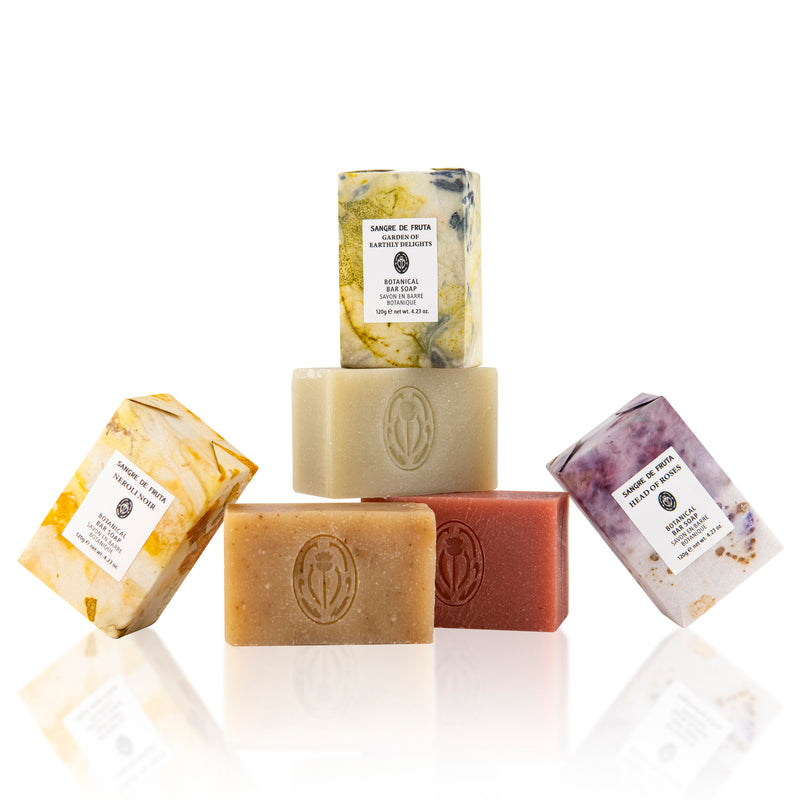This photograph features a meticulously arranged display of six bars of soap set against a pristine white background on a reflective white surface. The composition forms a small pyramid: three bars stacked at the base, one standing upright on top, and two more bars leaning against the structure from the left and right. 

Three of these bars are wrapped in elegant folded paper packages, adorned with labels. The top bar's label reads "Sangre de Fruta, Garden of Earthly Delights," with a black logo and additional text that says "Botanical Bar Soap" and "Savant" in French, along with the weight. The left bar is labeled "Neroli Noir," while the right bar, more purple in hue, reads "Head of Roses."

The unwrapped bars, showcasing their natural colors, include light brown, red, and dark yellow. The photograph captures the shadows and reflections created by this carefully balanced arrangement, adding depth and dimension to the white-on-white setting.